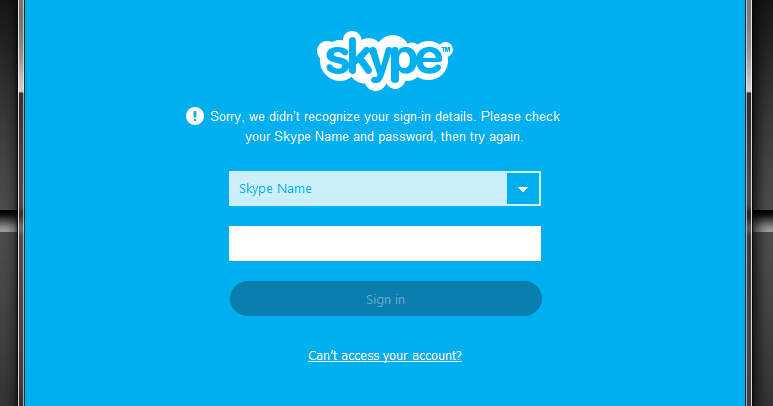This is a large, rectangular screenshot of a Skype login page, predominantly featuring a dark baby blue color scheme. At the top of the page, the Skype logo is prominently displayed. The logo consists of the word "Skype" with a trademark symbol, designed to resemble a cloud, with the letters matching the background blue and outlined in white.

Beneath the logo, an error message is prominently displayed within a circle containing an exclamation point. The message reads: "Sorry, we didn't recognize your sign-in details. Please check your Skype name and password, then try again." This is followed by a dropdown list currently set to "Skype name," suggesting users can select their login method. 

Below this dropdown is a field for entering the Skype name. The "Sign In" button, located beneath the input field, is dark blue, giving the impression that it has been pressed. The button's text is a dulled gray, likely indicating an error state that triggered the error message above.

Finally, at the bottom of the screenshot, there is an underlined, white link that reads: "Can't access your account?"